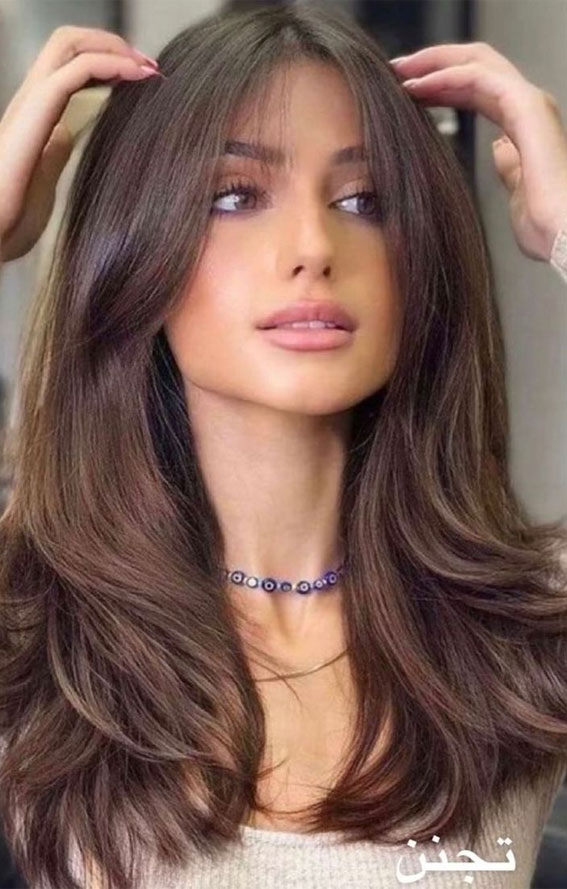The image, taken indoors, likely in a salon, showcases a color photograph of a female model or actress. She is situated in a setting that is partially obscured, with the background appearing blacked out. The focus is on her as she gazes off to the right, possibly into a mirror, with her hands gently stroking her freshly styled, long, soft, wavy brown hair, which features light blonde highlights. Her makeup is meticulously done, accentuating her large hazel eyes, long eyelashes, sculpted eyebrows, and pink lips. Around her neck, she wears a distinctive necklace featuring blue, white, and black beads with an intricate evil eye motif. She is dressed in an oatmeal-colored crop top or shirt, and the image captures her from the chest up. Notably, the bottom right corner of the photo contains white Arabic lettering, adding a unique cultural element to the scene.